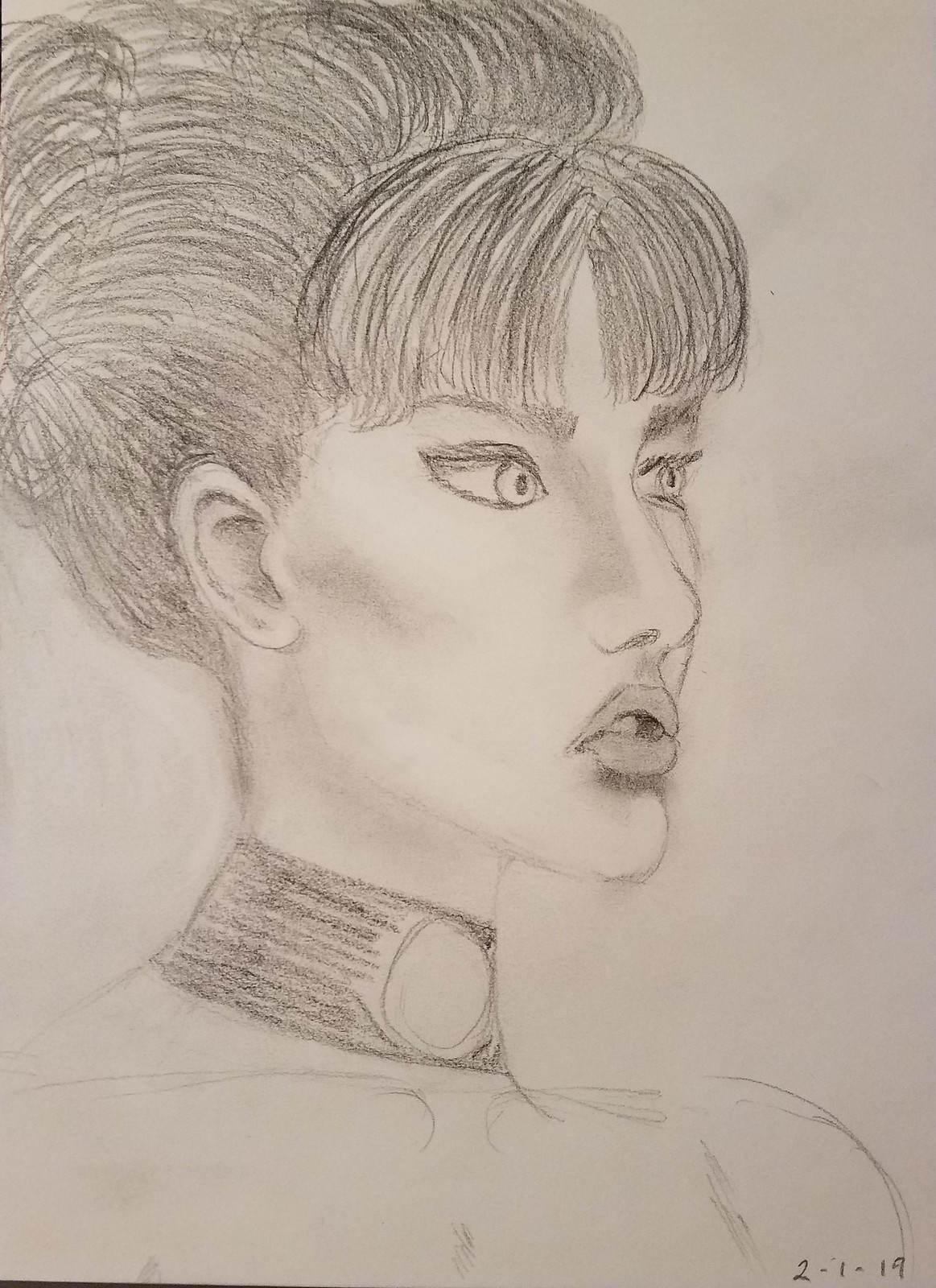The detailed pencil drawing features a close-up of a woman's face and upper torso, skillfully rendered on white sketch paper. The woman, adorned with a thick, black choker that showcases a prominent white circular medallion at its center, gazes off to the right side of the composition. Her long hair is elegantly pulled back into a voluminous bun, with soft bangs sweeping down to her eyebrows, parted slightly in the middle. Her wide eyes are full of life, and her slightly open lips add a touch of expression to her serene visage. The detailed shading extends to her neck and clavicles, marking the end of the primary focus area. The date "2-1-19" is inscribed in pencil at the bottom right corner, adding a personal touch to the artwork. The subtle, thin lines indicate her upper torso, blending seamlessly into the light gray texture of the paper, providing a refined and elegant finish to the portrait.